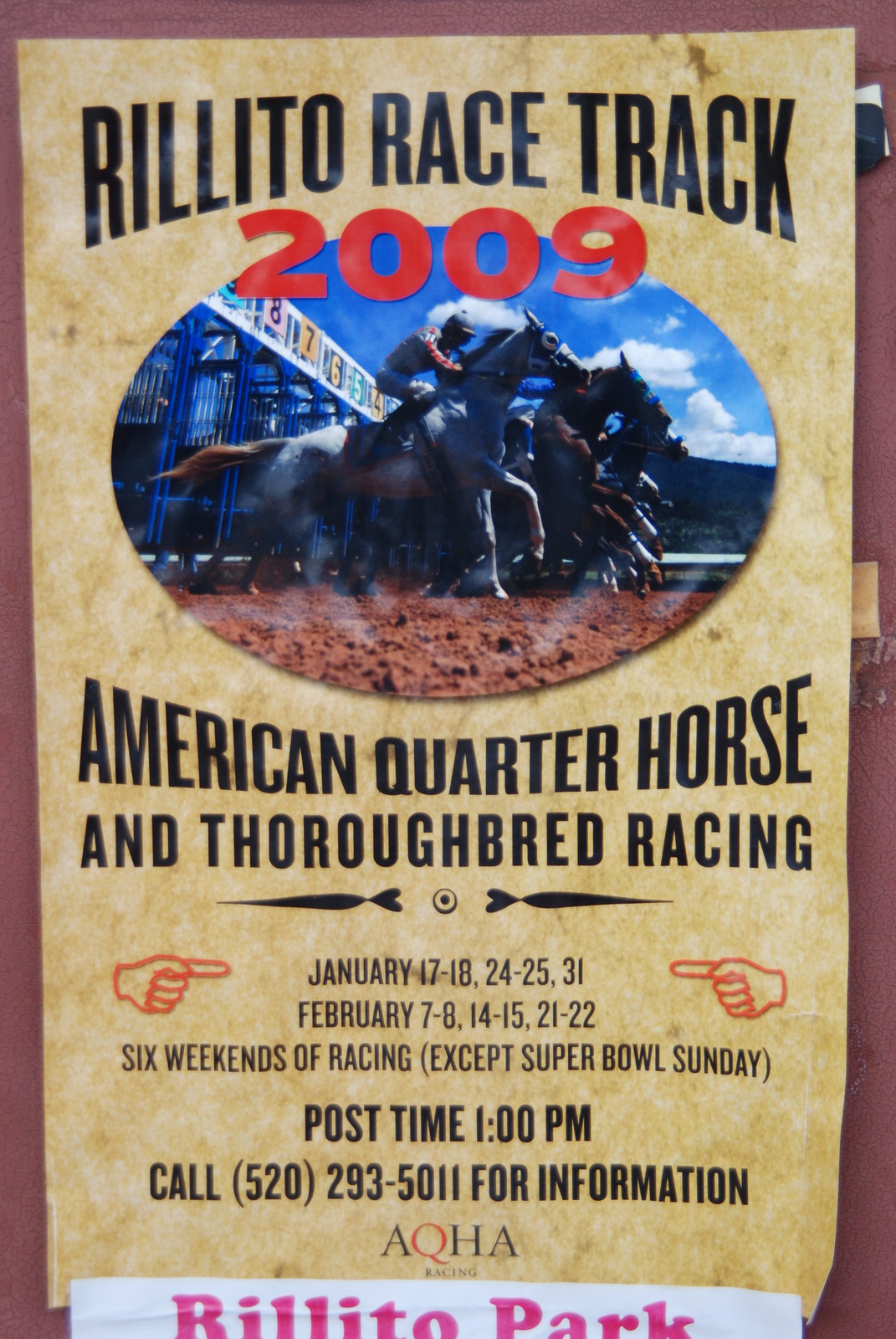This detailed poster for Relito Racetrack 2009 is mounted on a rich, dark-red background. The prominent top half of the poster features "Relito Racetrack 2009" with "2009" highlighted in vivid red against a circle backdrop. Within this circle, there is an evocative photograph depicting galloping horses with jockeys riding under a bright blue sky dotted with white clouds. The horses race on a rich brown track, adding a dynamic element to the imagery. Below this striking visual, the text announces "American Quarter Horse and Thoroughbred Racing", followed by multiple racing dates: January 17-18, 24-25, and 31, February 7-8, 14-15, and 21-22, noting that these six weekends of racing exclude Super Bowl Sunday. Illustrations of fingers point to the dates for emphasis. Additional details inform that post-time is at 1 PM and provide a contact phone number: 520-293-5011. At the very bottom, against a white background, the affiliations "AQHA" and "Relito Park" are highlighted in pink letters, underscoring the venue and race organization.